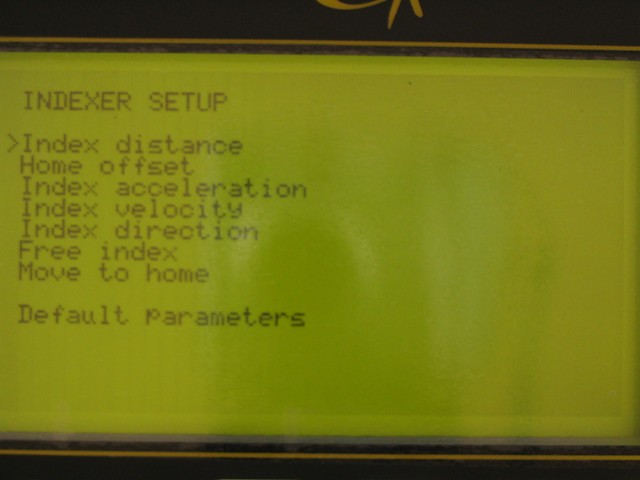In this image, an individual is observing a screen, which could be a computer, tablet, or handheld device, displaying a user interface titled "Indexer Setup." The screen has a yellow background, with all text appearing in black. An arrow points towards the "Index Distance" parameter on the interface. Below this heading, the following options are listed from top to bottom: "Home Offset," "Index Acceleration," "Index Velocity," "Index Direction," "Free Index," "Move to Home," and "Default Parameters." Above these options, a partial gold-colored drawing is visible, though its details are unclear. There is a faint reflection on the screen that suggests the shadow of a person standing before it. The screen is small and rectangular, casting doubt on whether the device is a personal computer.